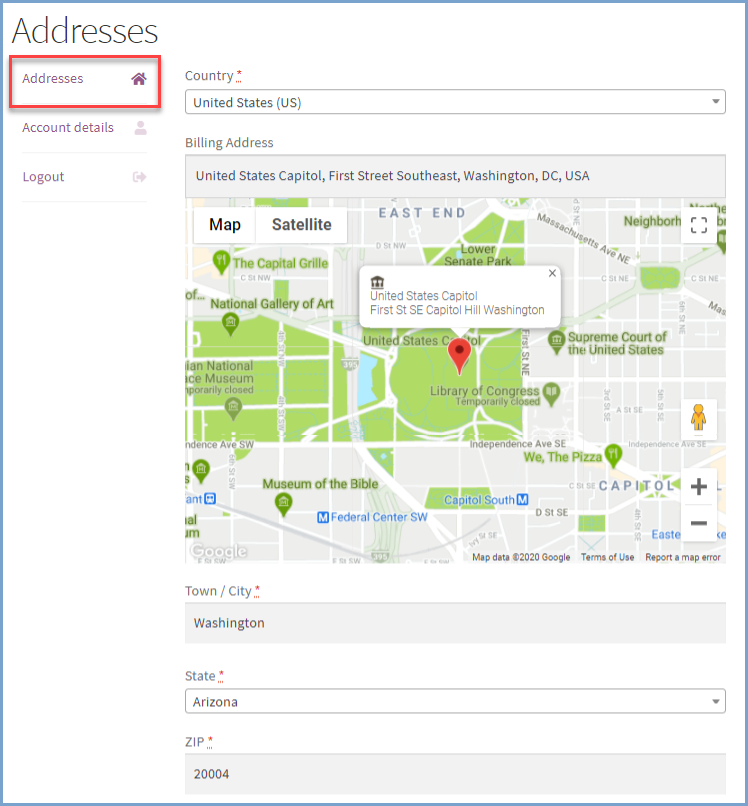The upper left corner prominently displays the word "Addresses" in large text. Below this, another address is shown in a smaller, burgundy-colored font. A red box highlights this section, and beneath it, there is a small house emoji. Nearby, "Account Details" is written in red, but it is faded. Next to it, there is a person icon and below that, a "Log Out" option with another emoji.

To the right, directly across from the "Addresses" section in the left-hand column, you will find "Country" marked with a red asterisk, indicating that it is a mandatory field. Currently, "United States" is selected. Beneath this, the "Billing Address" is listed as: "United States Capitol, First Street, Southeast, Washington, DC."

A map is displayed with green areas representing grassy terrains, and blue areas representing bodies of water. In the center, a red pin marks "United States Capitol" and repeats the address. You can close this map at the top right corner. The map also features various green pins highlighting historic places around Washington, DC, like the Library of Congress, Museum of the Bible, and "We the Pizza." Blue pins indicate metro stations. The map interface includes a white-labeled zoom-in feature in a blue box at the top right, with plus and minus signs below it for scaling.

Further down, fields are available to input the town or city, currently set to "Washington." Below that is the state field, marked with an asterisk and showing "Arizona," and finally, the ZIP code field, currently set to "20004."